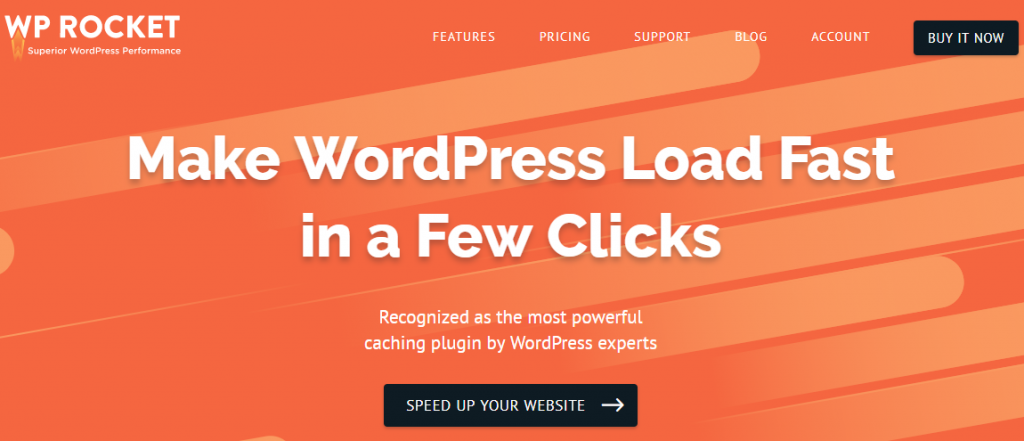This is a left-to-right horizontal image, resembling an advertisement typically seen in emails or on web pages. The background features various shades of orange with lighter, rounded rectangular lines crossing it horizontally. In the upper left-hand corner, the text "WP Rocket" appears in white, followed by additional information. 

In the center-right section, there are menu options written in white: "Features," "Pricing," "Support," "Blog," and "Account." Adjacent to these, a black box with white letters prominently displays the call-to-action "Buy It Now."

At the heart of the advertisement, a bold white headline declares, "Make WordPress Load Fast." Directly below this, another line reads "in a few clicks." Following this is a white subheading that says, "Recognized as the Most Powerful Caching Plugin by WordPress Experts."

Towards the bottom, a black rectangular box with all-uppercase white text commands, "SPEED UP YOUR WEBSITE," accompanied by a white arrow pointing to the right.